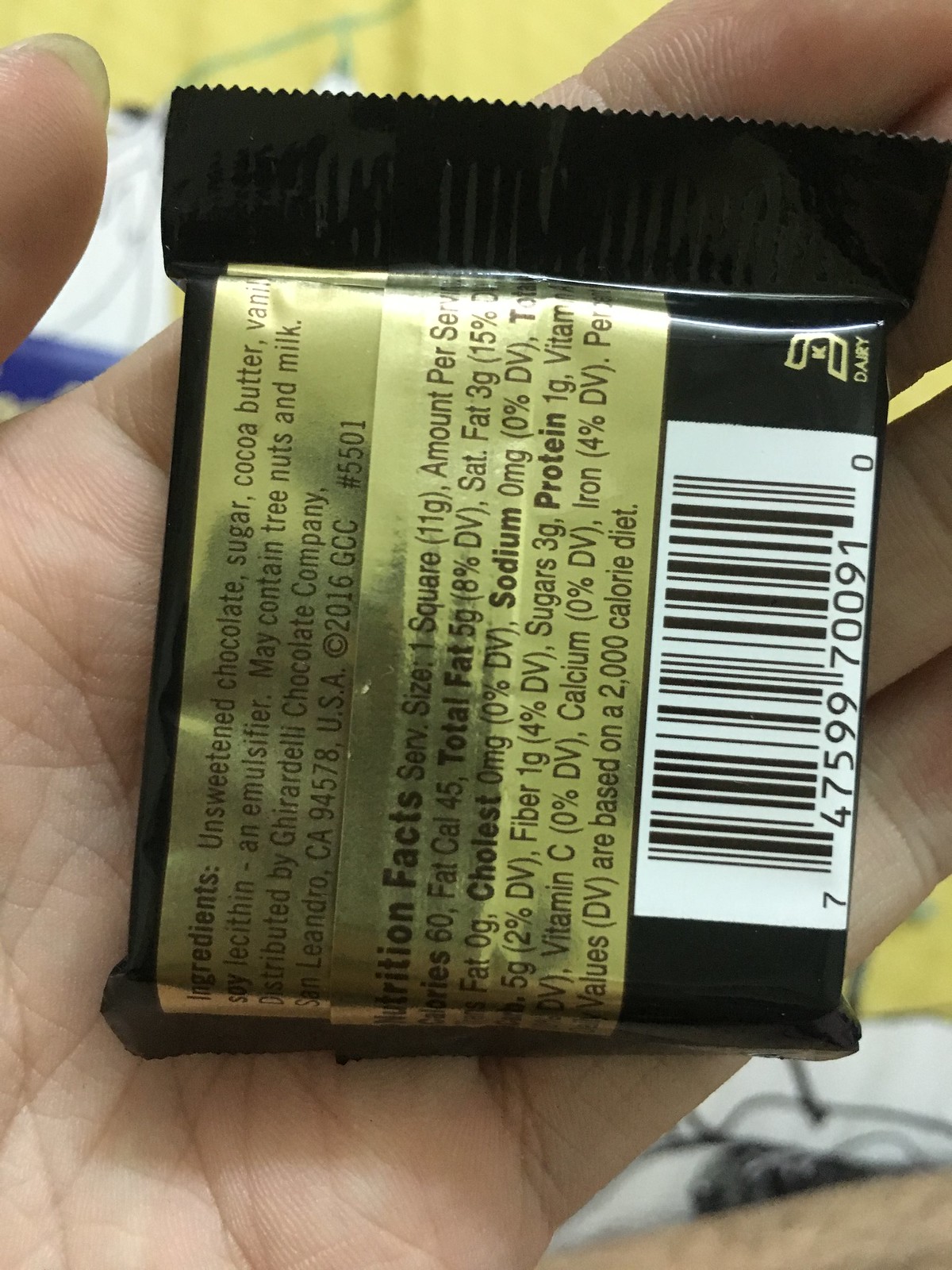A detailed view of the back of a sealed snack package is prominently displayed. The ingredients are clearly listed, including chocolate, sugar, cocoa butter, and vanilla, with a note that the product may contain traces of nuts and milk. Nutrition facts are comprehensively provided, even listing items with 0% values, giving a thorough yet slightly overwhelming impression. Additionally, a barcode is visible, indicating it's a single-serving product, roughly the size of a palm. Notably, the front of the package remains hidden, obliging an assumption that it is indeed a single-serving snack. The bottom-right corner is marked with "Dairy," reinforcing the inclusion of milk in the ingredients. Despite its small size, this little snack promises a hint of sweetness, perfect for a quick treat.